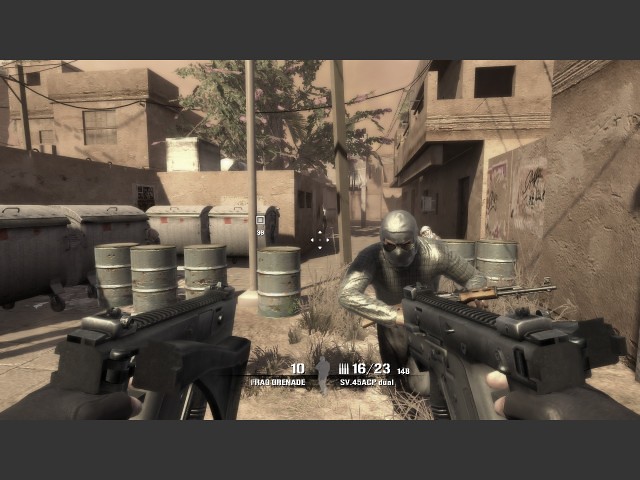A still photograph captures the first-person perspective of a shooter video game set in a scorching, arid environment. The scene, painted in muted and grayscale tones, mimics the aesthetic of games like Halo. From the player’s viewpoint, two guns are prominently aimed at an unseen opponent in the foreground. The background is cluttered with industrial elements: six gray barrels are aligned haphazardly near a couple of trash dumpsters. Surrounding these objects are dilapidated structures, seemingly constructed with a rudimentary, mud-daub technique, contributing to the game's gritty atmosphere. In the distant background, a lone tree is visible, emerging between two weathered buildings, adding a touch of life to the otherwise desolate scene.